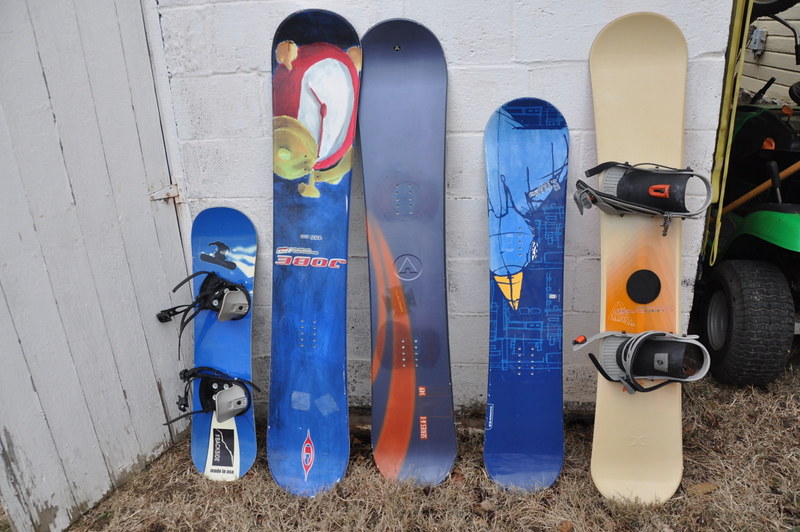This is an outdoor photograph featuring five snowboards leaning against a white-painted brick wall with large bricks. The ground below is covered in brown, dead grass, and there's a wooden door situated next to the wall, painted white.

From left to right, the first snowboard is a small, dark blue children's board featuring a graphic of a snowboarder jumping off a hill. Its feed securing clasps are attached to the top of it. Beside it, the second snowboard is a dark blue board with multiple blue tones and an orange V and an A on it. It stands as one of the taller boards. The third snowboard has a striking midnight blue coloration with dark blue lines and a small yellow triangle where the lighter blue meets the darker blue. Next to it is a dark blue snowboard marked with "380J," featuring a vibrant red alarm clock graphic with golden bells on the face. It stands as the tallest board. The final snowboard on the far right is a cream-colored adult board with feet securing clasps, identified by its beige hue with an orange middle section and a distinctive black circle. The picture also captures a green tractor with a visible black wheel in the corner.